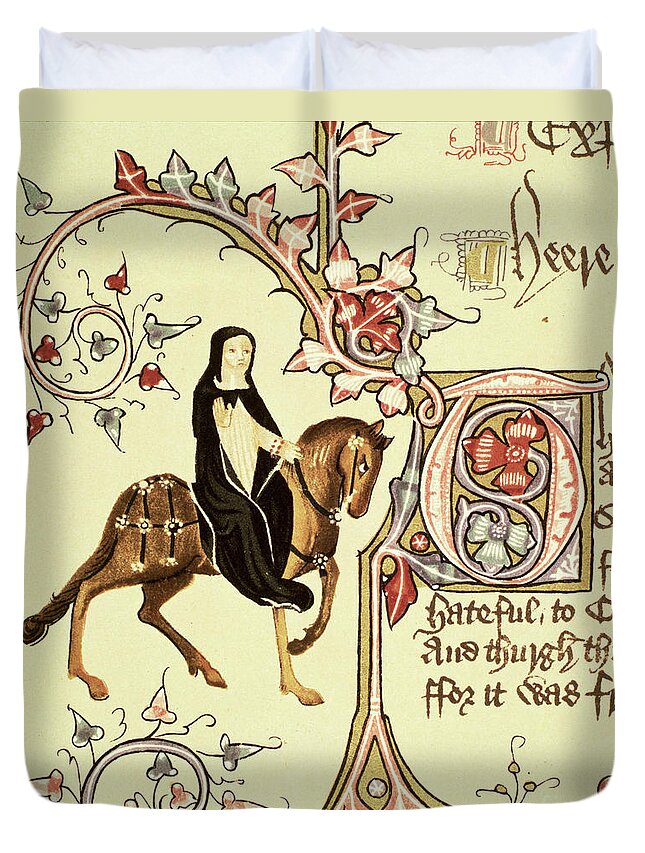The image is a detailed close-up of a satchel or bag against a very light off-white, almost yellowish background. The bag contains two white, pillowy objects at the top, suggesting they are inside it. The background features intricate design elements, including fancy red medieval-style writing that is difficult to read. A light brown vine curls around the middle of the image, adorned with red and gray flowers, adding an animated touch. To the left of the image is a depiction of a woman in a long black dress, riding a brown horse. The scene evokes an old-fashioned, almost medieval feel, with the woman appearing somewhat like a nun from the 1800s. The artistic rendition is set on yellowish paper, complemented by delicate flowery branches and stems, giving it a very ancient and delicate appearance. The color palette includes red, white, yellow, and greenish hues, contributing to its intricate and delicate style.